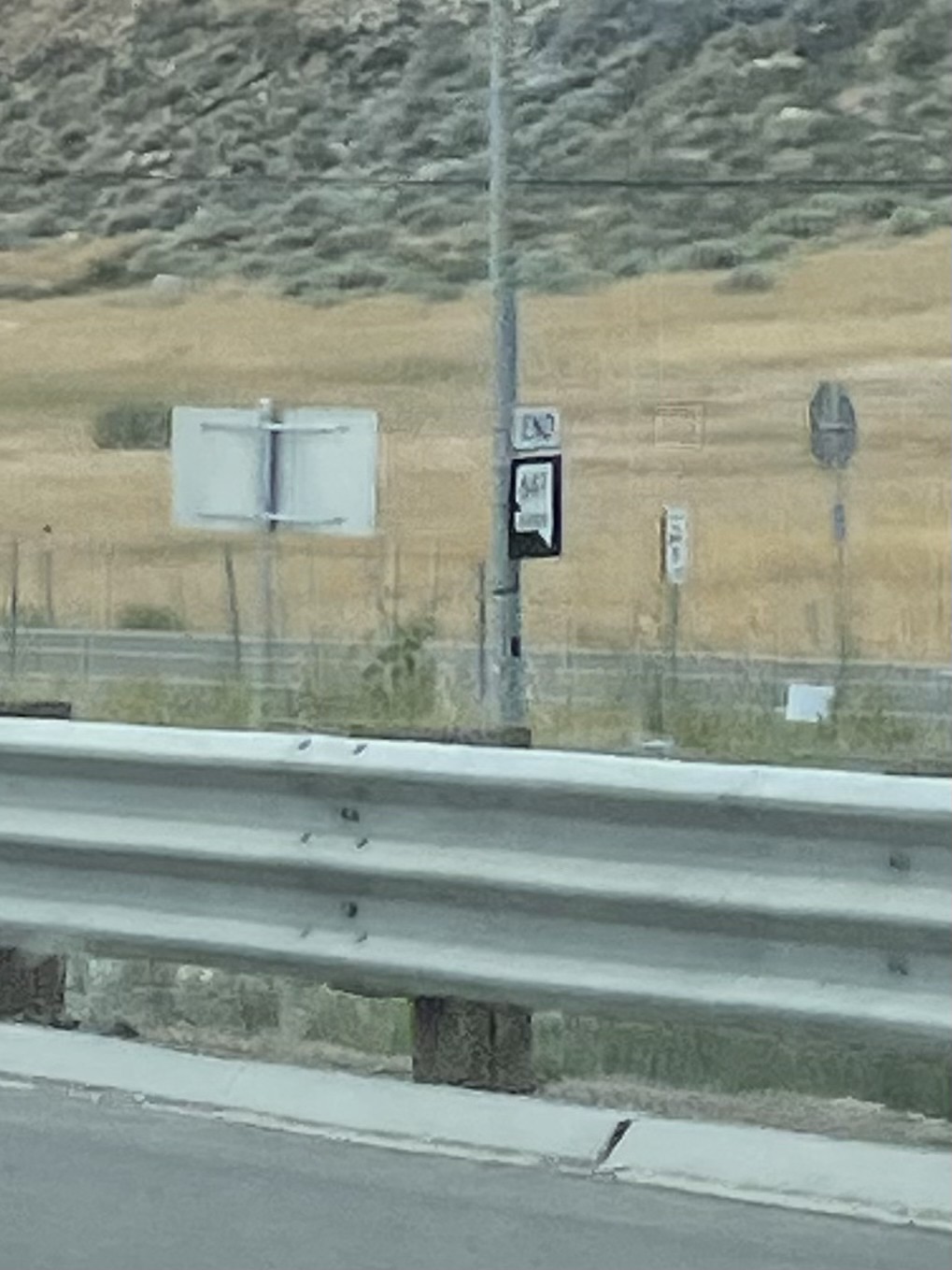This photograph captures a scene on the side of a remote highway. The foreground prominently features an asphalt road bordered by a large metal barrier. Adjacent to the road and barrier is a curb, which separates the roadside from a grassy island filled with greenery in the center of the highway. In the midground, the road's opposite lane runs horizontally across the image, marked by various signs including one that reads "End" and a stop sign. The backdrop of the image showcases a vast expanse of dried grassland, interspersed with clusters of gray boulders scattered across the horizon. The scene conveys a sense of isolation and the stark beauty of the natural landscape on the outskirts of the highway.